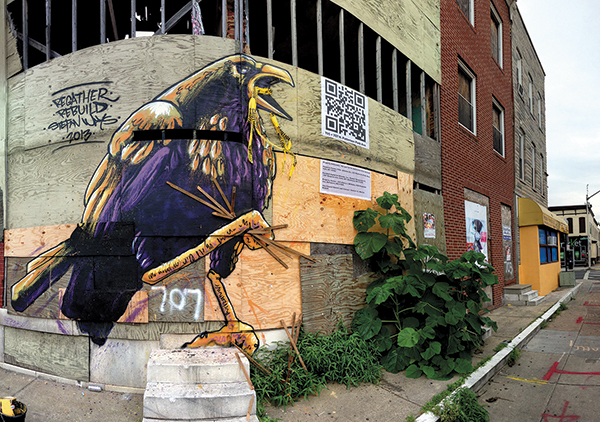This photo captures a uniquely adorned corner lot building, which is currently boarded up with wood planks and wooden side paneling. The corner of the building is slightly rounded, and one side features an additional brick wall. Prominently displayed on the building is an intricate mural of a crow. This crow features vibrant purple feathers on its lower body, a striking gold head and beak, and orange-gold accents on its backside. The bird appears to be holding a bundle of sticks. Additionally, the mural includes a QR code for passersby seeking more information and the inscription "Regather Rebuild 2013".